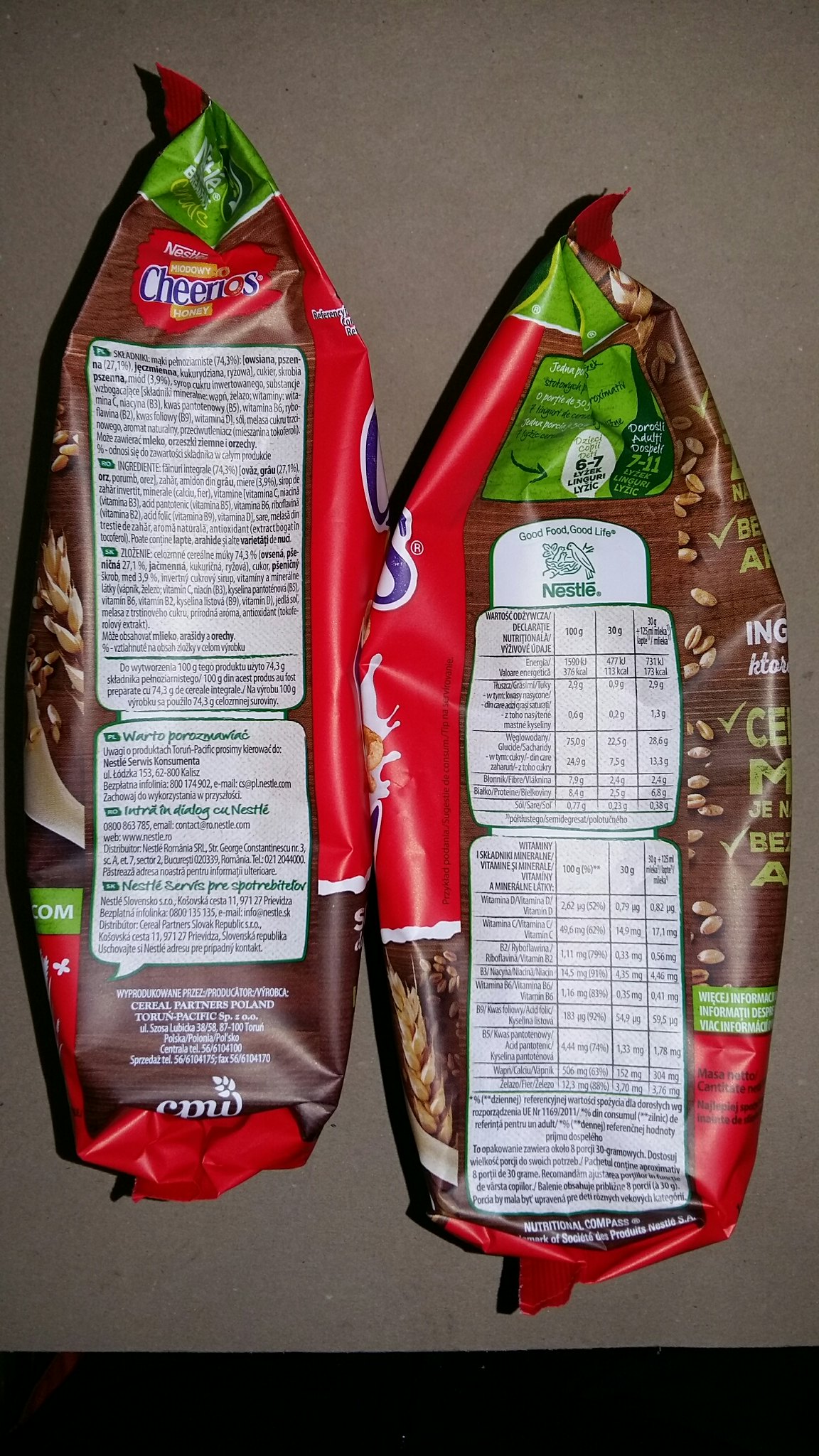The image depicts two retail packages of a cereal treat, prominently branded with the Cheerios logo. Both bags are predominantly red with distinctive brown and green accents. The package on the left features "Cheerios" and the word "Honey" at the top, suggesting a honey-flavored variant. The bag also includes an extensive area of text which likely provides preparation instructions. The right package sports a green area at the top bearing the text "Good Food, Good Life" alongside the Nestle logo, which features a green bird's nest. Below this, various nutritional details are given for different serving sizes, including 100 grams, 30 grams, and 30 grams with milk. Although the text is partially illegible, it indicates the high-calorie nature of the treat. Both packages exhibit a brown backdrop adorned with small seeds and a splash of milk on the image, hinting at a convenient breakfast or snack item. The overall design and details suggest a fusion between traditional Cheerios cereal and a more indulgent, possibly honey-flavored, treat.